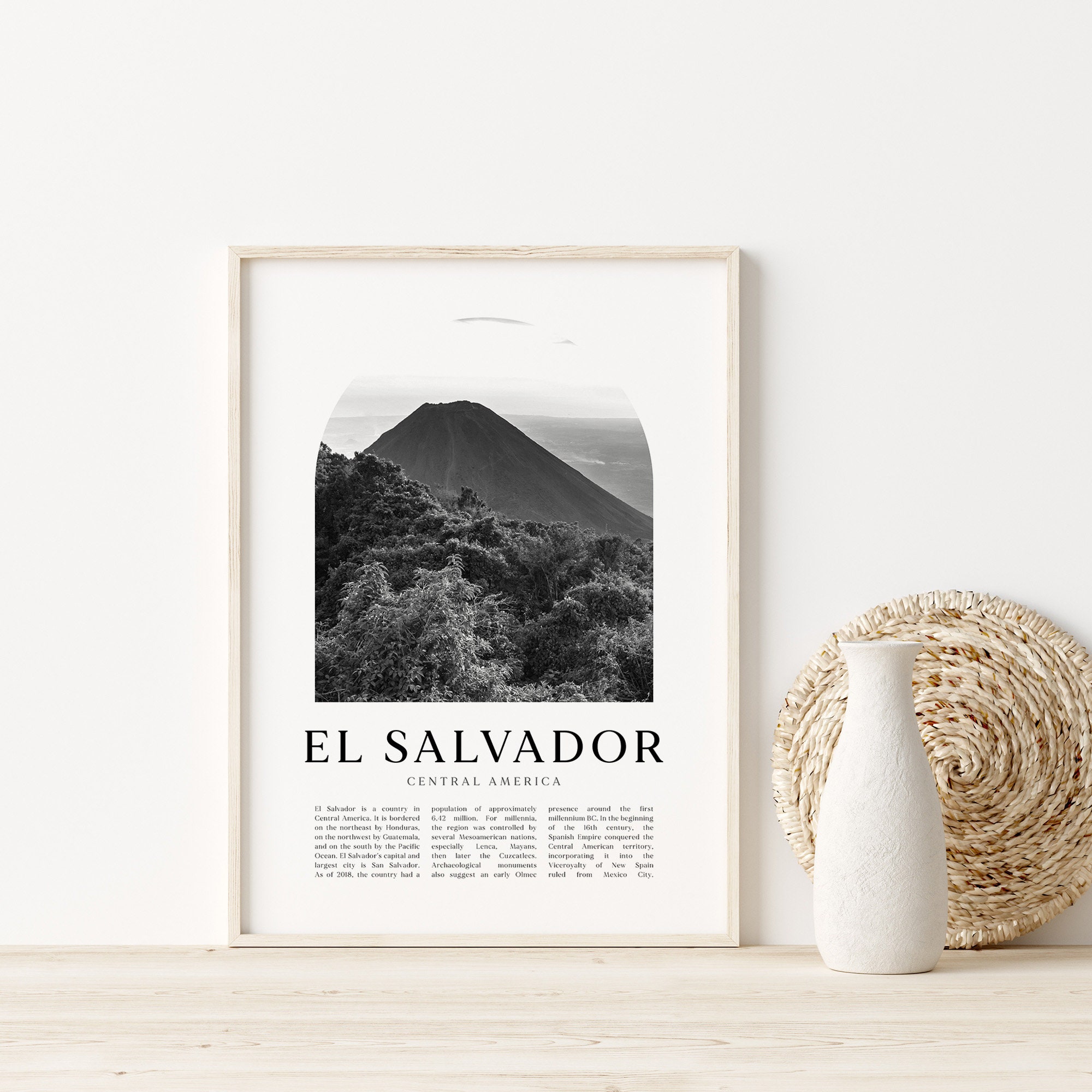The image features a section of an elegantly styled home interior, showcasing a light greenish-white wooden table (or shelf) against a white wall. Central to the décor is a framed print with a beige or light wood-colored frame depicting a black and white scene of a mountainous region in El Salvador, Central America. The image features dense foliage, a line of water in the background, and a bright white skyline above. Beneath the image, the print includes the text "El Salvador, Central America," followed by three paragraphs of smaller text that provide some information about the place. To the right of this framed artwork, there is a tan, textured, crocheted or woven round piece leaning against the wall. In front of this artistic piece, there is a white, textured clay pot that resembles an old milk jug, suggesting it could be used to hold flowers. These items are positioned neatly on the cream-colored shelf, contributing to the serene and aesthetically pleasing arrangement.